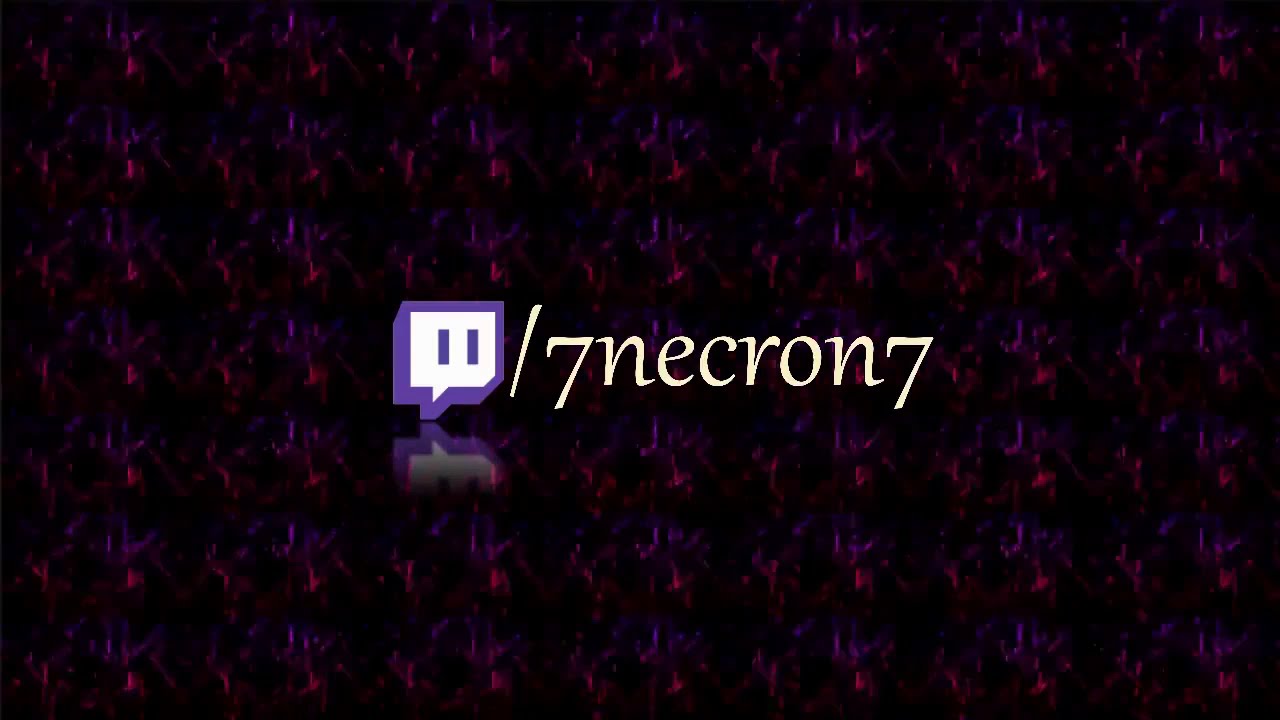The image features a horizontally stretched rectangular background with a repetitive, pixelated pattern in shades of purple, light red, and black. The pattern gives off a smoky or magic-eye illusion, adding depth and texture to the scene. In the center of the composition, the Twitch logo, which resembles a speech bubble with two vertical lines, is prominently displayed in a purple and white color scheme. The words "7NECRON7" are written in a white, serif font, both within and beneath the speech bubble, with a forward slash preceding the first "7." The Twitch logo appears to be reflected below, adding a mirrored effect. The vivid background design complements the logo and text, making for a visually striking header suitable for online use.